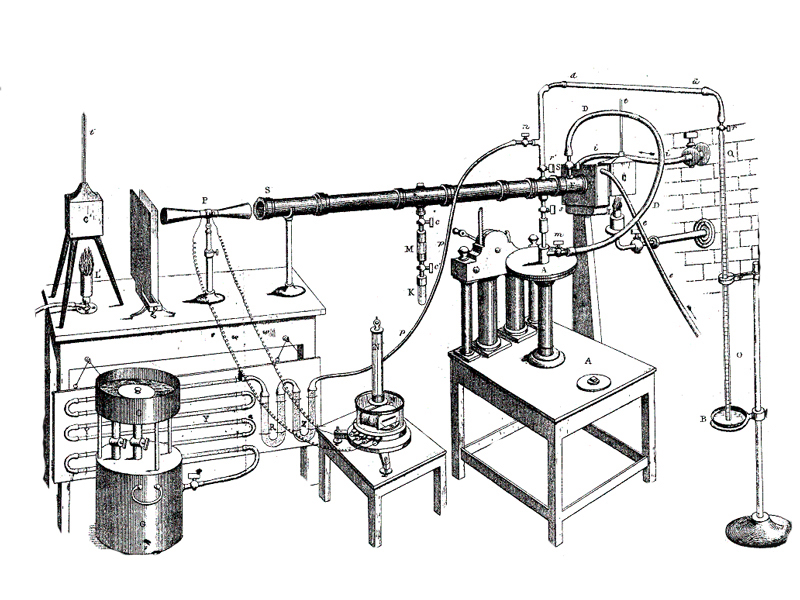This image is a detailed black-and-white technical illustration, likely sourced from the mid-1850s, depicting Tyndall's experiment related to the absorptive power of gases in the atmosphere, a foundational study for understanding the greenhouse effect. The landscape-oriented sketch features a plethora of metal machinery and tubular devices distributed across multiple tables of varying heights.

On the left side, there's a countertop with several apparatuses on top of it. In front of this table stands a cylindrical object, with a solid base, an open middle section, and a top lid, possibly silver or gray in the original context. To the right of this countertop is a stand supporting a long metal tube that extends rightward, connecting to another apparatus across the room. This apparatus, likely part of a complex mechanism, is supported by its own stand and features multiple tubes that extend upward, curl, and then connect to yet another device sitting on a smaller table in the right section of the frame.

Between the cylindrical device and the smaller table, there is an additional table holding an apparatus with a rounded base and an upwardly extending tube. Behind this setup is an arching tube that descends to a circular base on the right. In the bottom right-hand corner, another circular base supports a vertical rod. The background showcases an implied brick wall in the upper right section, suggesting an indoor setting for this historical scientific setup.